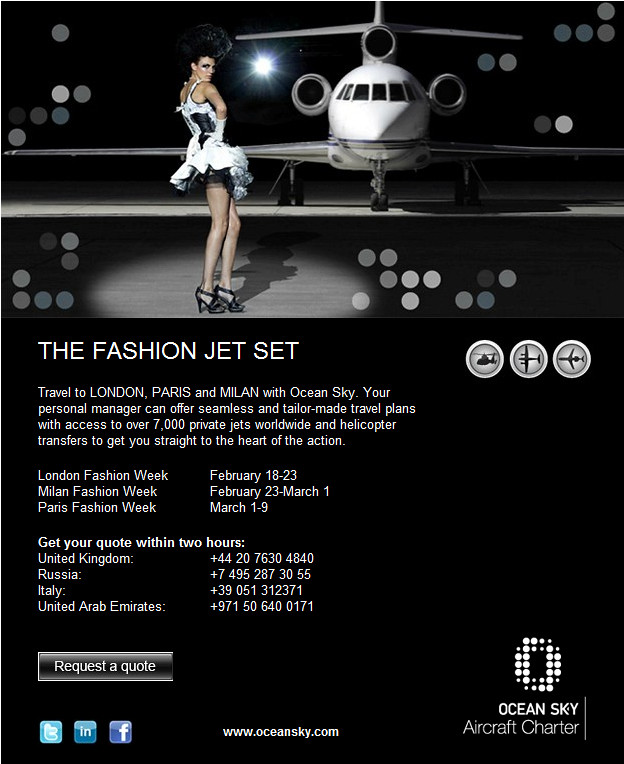This poster for Ocean Sky Aircraft Charter features a high-fashion theme targeted at jet-setting travelers attending international fashion weeks. The upper right section of the poster, set against a black background, prominently displays a sleek white private jet—likely a Learjet or Bombardier—on the ground, with three engines, a tail fin, and wing structures. In the foreground stands a woman in an elegant, fluffy cocktail dress with a sleeveless, strapped design. She wears black stockings, high heel shoes, and a distinctive headdress over her black hair, staring confidently forward. 

The poster's central section showcases bold white text that reads, "The Fashion Jet Set." Beneath this, smaller white text elaborates on the exclusive travel offer: "Travel to London, Paris, and Milan with Ocean Sky. Your personal manager can offer seamless and tailor-made plans with access to over 7,000 private jets worldwide and helicopter transfers to get you straight to the heart of the action." It provides detailed information about the upcoming fashion weeks: London Fashion Week (February 18-23), Milan Fashion Week (February 23-March 1), and Paris Fashion Week (March 1-9). 

Further, the text encourages readers to "Get your quote within two hours," and provides contact numbers for the United Kingdom, Russia, Italy, and the United Arab Emirates. Instructions to "Request a quote" are included, accompanied by logos for Twitter, LinkedIn, and Facebook on the lower left. At the bottom center, the poster shows the Ocean Sky logo—white dots on a black background—with the text "aircraft charter" underneath. The web address, www.oceansky.com, is prominently displayed, ensuring viewers know where to go for more information.